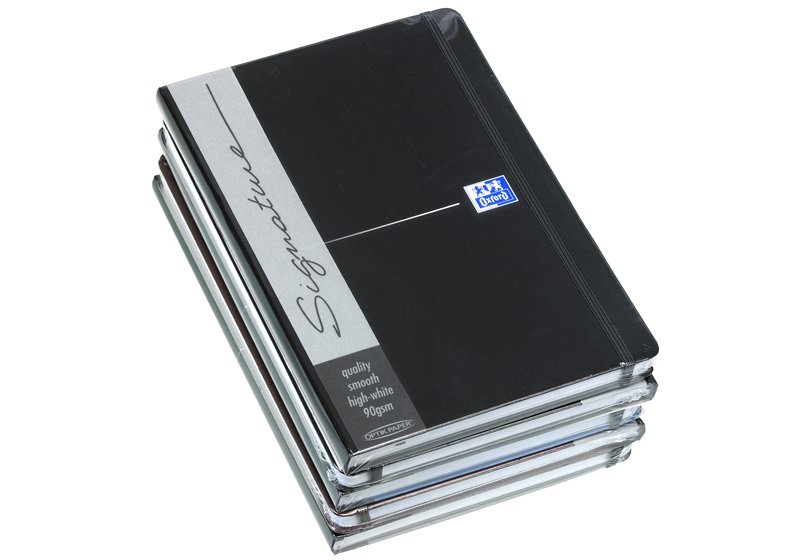This image features a neatly stacked set of five sleek, black journals positioned against a pristine white background. Each journal boasts distinct characteristics: along the left side, the word "signature" is elegantly scripted in cursive within a gray vertical strip. The cover of the topmost journal prominently displays the label "quality smooth high white 90 GSM optic paper" in a square at the bottom corner. A striking blue and white sticker, bearing the brand name "Oxford," adorns the middle right of the cover, intersected horizontally by a subtle silver line. Additionally, a sturdy fabric band, akin to a shoelace, runs vertically along the right side, possibly serving as a clasp to keep the journal securely closed. The minimalist white background accentuates the refined and sophisticated design of these high-quality journals, making them perfect for capturing life's memorable moments, whether joyous or sorrowful.